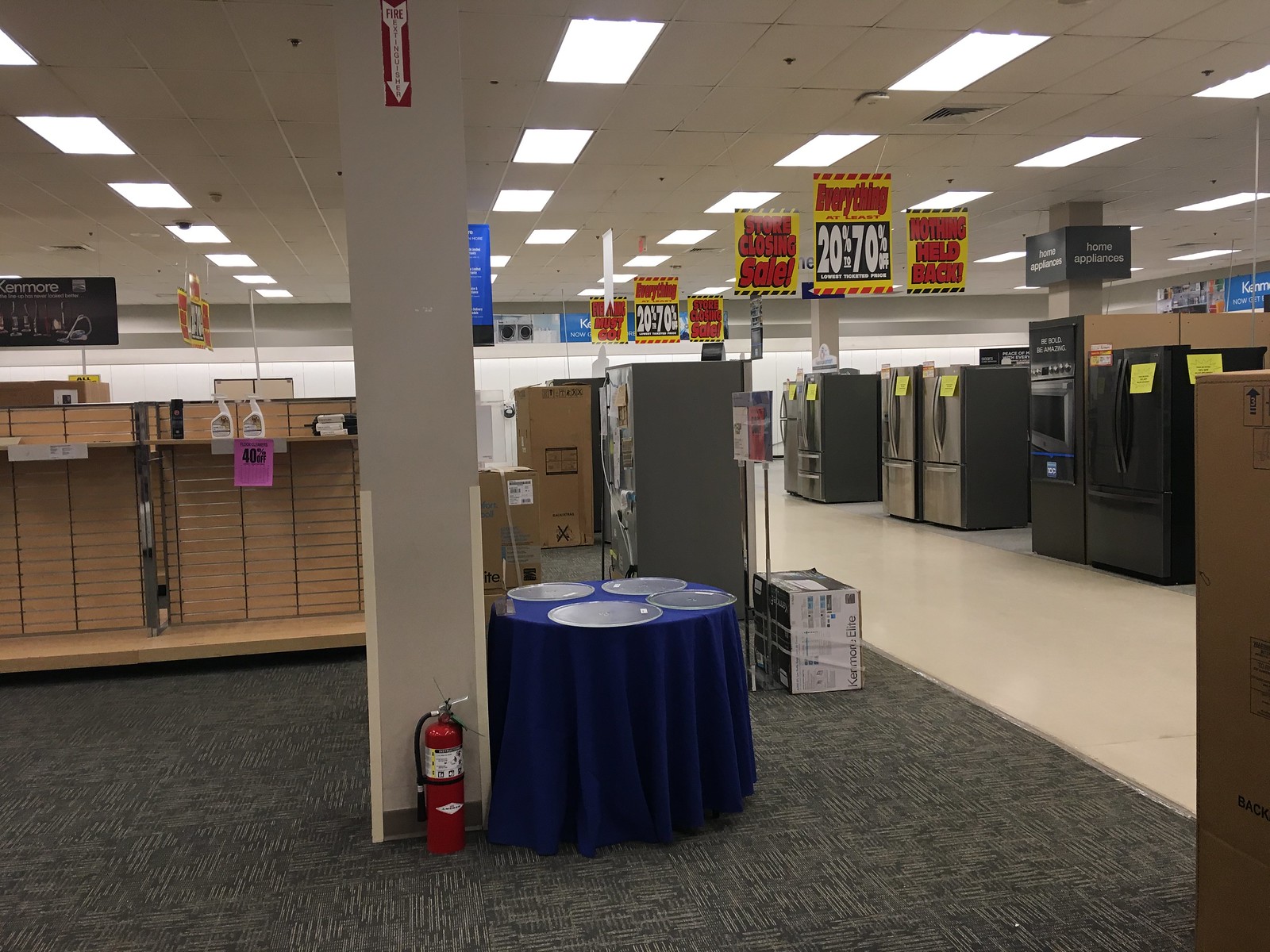The image depicts the interior of a department store, specifically the appliance section, during a store closing sale, signaled by numerous red and yellow signs hanging from the white paneled ceiling. These signs, featuring white numbers on black borders, announce a massive liquidation with everything discounted by 20 to 70 percent, emphasizing phrases like "Store Closing Sale," "Everything Must Go," and "Nothing Held Back." On the left-hand side of the image, there are mostly empty shelves with just a few bottles left. In the center, there's a blue tablecloth-covered table with four empty glass plates, possibly previously used for samples, standing on a gray carpeted floor next to a fire extinguisher. The aisle divides the scene, leading to the right-hand side which showcases the home appliances section, identifiable by a blue "Kenmore" sign. This area contains various large kitchen appliances like silver and black refrigerators and ovens, all marked with yellow sale signs. The store is bathed in fluorescent light, highlighting the sparsity and vacancy typical of a closing sale environment.